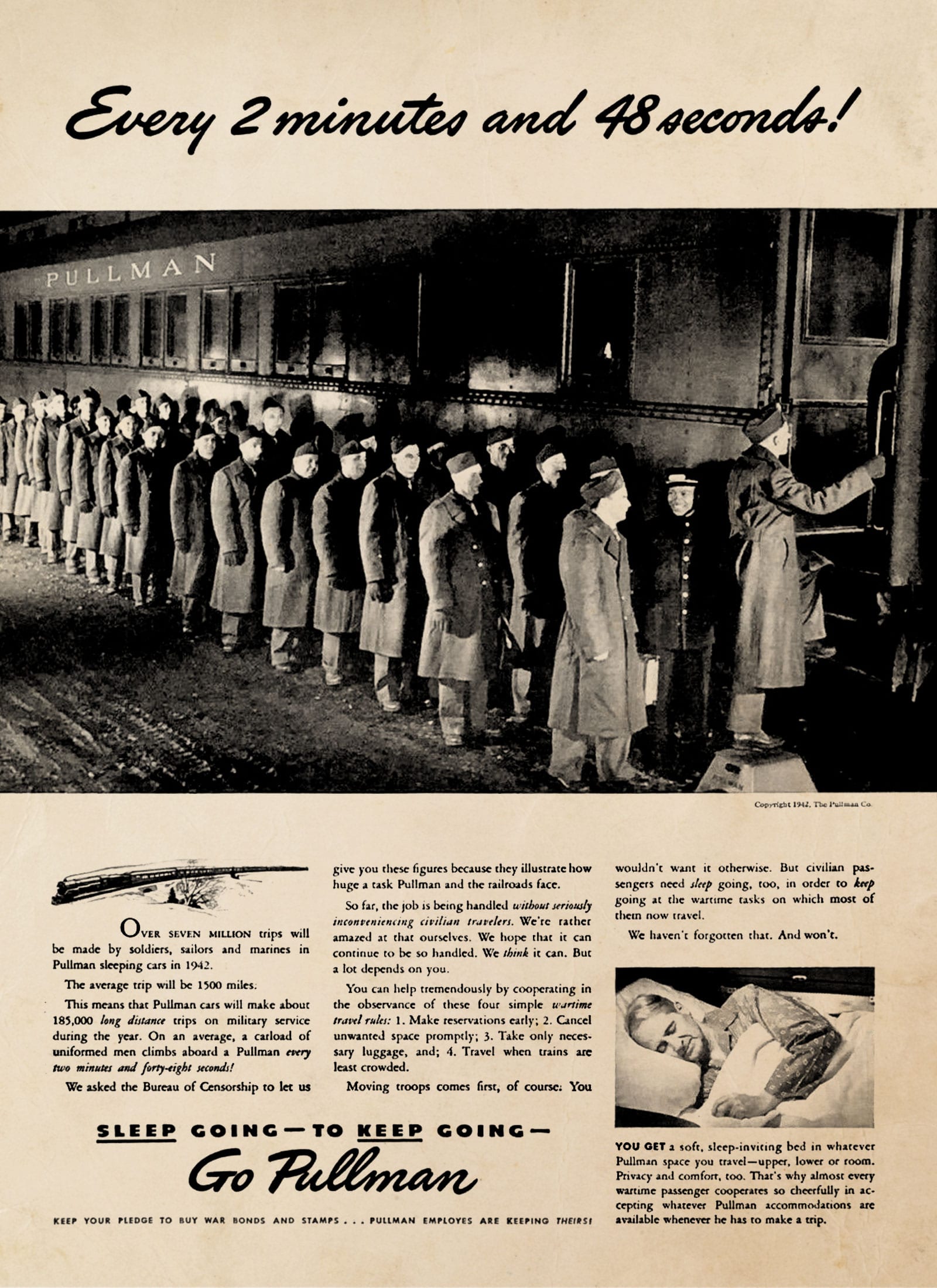This vintage advertisement, likely from a 1942 magazine or newspaper, promotes Pullman sleeping cars used in military transportation. The central image, rendered in black and white, depicts several soldiers lined up to board a Pullman train. One soldier is already stepping aboard. The backdrop, a pinkish-tan, old-timey paper, enhances the nostalgic feel of the ad. At the top, the headline, "Every two minutes and 48 seconds," underscores the frequency of these military train journeys. Below the photo, the text highlights the extensive use of Pullman cars by soldiers, sailors, and Marines, estimating over seven million trips covering an average distance of 1,500 miles each in 1942. The advertisement emphasizes the crucial role these sleeper cars play in moving troops, ensuring that military personnel can rest en route to their destinations. A smaller image to the right shows a woman resting peacefully in a bed, symbolizing the comfort provided by Pullman cars. The ad concludes with a patriotic appeal: "Sleep going to keep going. Go Pullman. Keep your pledge to buy war bonds and stamps, Pullman employees are keeping theirs," and advises civilians on how to assist with wartime travel efforts by making reservations early, canceling unwanted space, taking minimal luggage, and traveling during less crowded times.